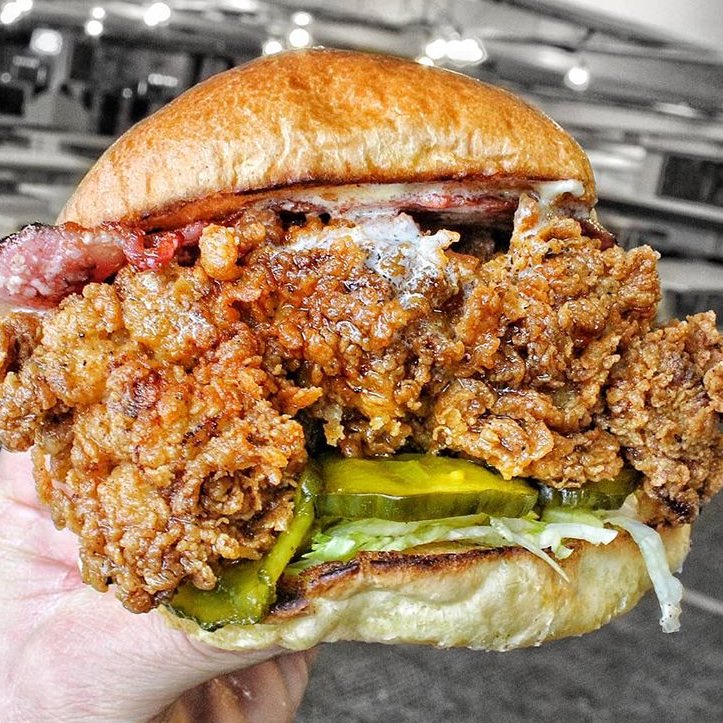This is a photograph showcasing a tantalizing honey butter burger. The burger appears impressively large and exudes a crispy, crunchy texture that suggests either fried chicken or beef as the patty. The sandwich is layered with thick slices of savory bacon, crisp pickles, and fresh lettuce, completed with what seems to be a slice of white cheese. The entire creation is nestled in a perfectly toasted brioche bun, golden and glossy.

A hand, visibly gripping the burger, is the only part of the person shown in the photo. The background sets the scene in a kitchen environment, identifiable by countertops positioned just beneath the burger. There’s a hint of digital enhancement, suggesting the burger might have been photoshopped into the hand and the kitchen backdrop, adding to the surreal and tempting visual appeal.